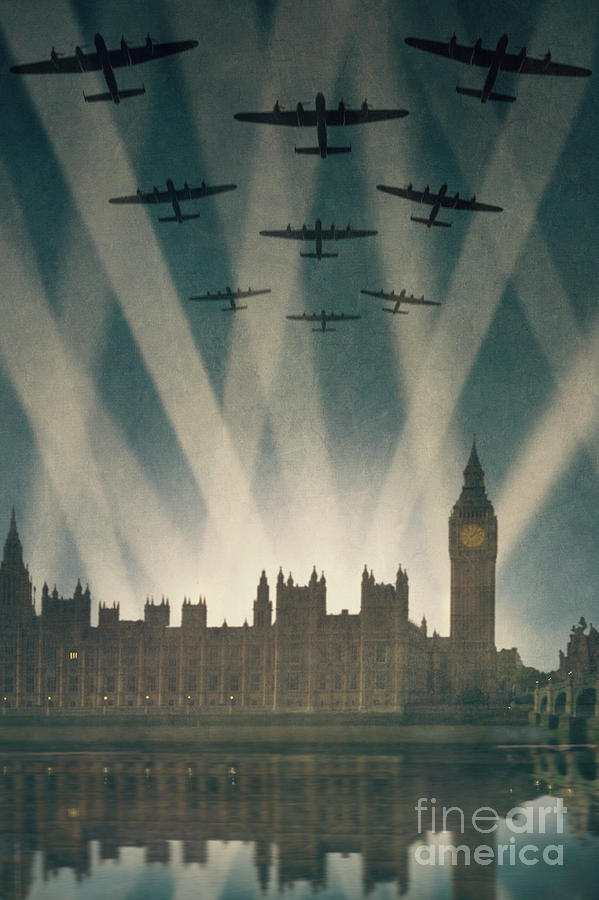The image is an artist's drawing depicting a dramatic scene from World War II, featuring the iconic Houses of Parliament and Big Ben situated on the riverbank, with their dark brown structures clearly visible. In the lower quarter of the image, the buildings reflect into the water, creating a mesmerizing mirrored effect. The backdrop is a very dark blue sky, illuminated by narrow, bright searchlights that emanate from behind the buildings, casting white beams that fade slightly as they extend upward. Silhouetted against the sky are nine dark planes, arranged in a loose formation of three rows of three, with each plane having two propellers on each wing. This haunting image, which blends a sense of historical depth with artistic interpretation, features the faint white overlay text "fine art america" in the bottom right corner, with 'fine' in thin letters and 'art' and 'america' in bold. The overall composition evokes a sense of wartime tension and atmospheric intrigue.